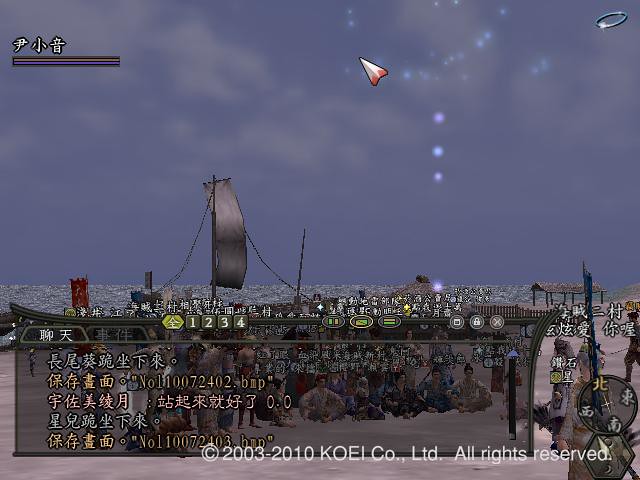This image appears to be a screenshot from a video game, featuring Chinese text in the bottom left corner. The scene is dominated by a picturesque sky above a serene body of water. A sailboat is partially visible, with its central sail and a long rod extending backward, adorned with a reddish flag. A translucent, light-colored text box typical in video games overlays part of the image. In the background, behind the text box, several people are seen sitting on a sandy beach, adding a touch of life to the tranquil setting.